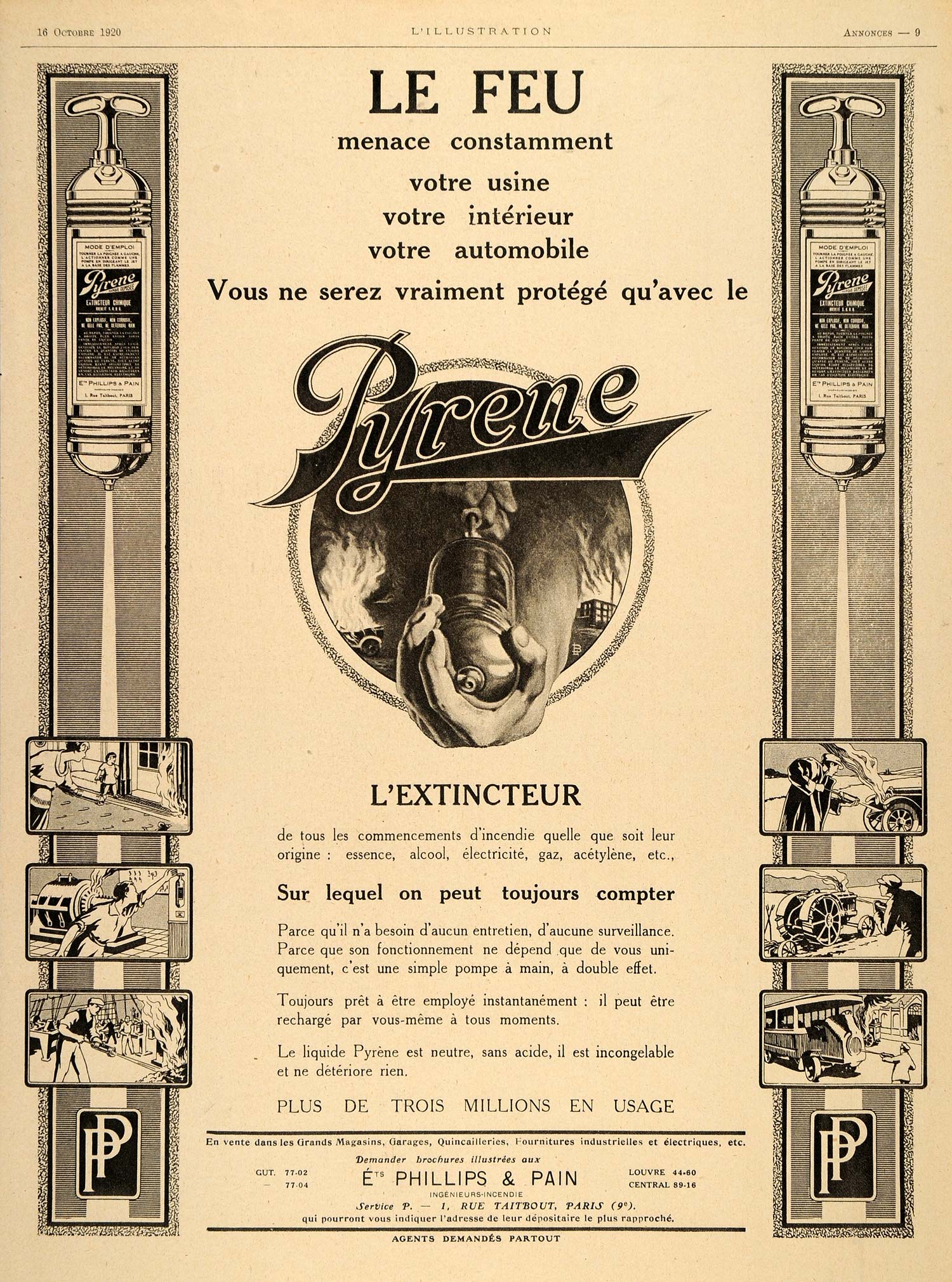This image is a detailed illustration of an advertising flyer from the 1920s, featuring aged, brownish-yellow paper and French text. At the top of the flyer, small print identifies it as an illustration, with "ANNANCES 9" noted on the right side, and a date in the upper left. Centered prominently in bold letters is the word "LEFEU." Below this header is a logo depicting a hand holding a cylindrical fire extinguisher within a circle, accompanied by the brand name "Pyrene." The central focus of the advertisement is on this hand-held fire extinguisher, described in the accompanying text as a vital household safety tool. The bottom section lists the company name and address, providing additional details about the manufacturer.

Flanking the main illustration are smaller images: on each side, at the top, there is a depiction of the cylindrical fire extinguisher, complete with a handle and spout. Further down on either side, there are three sequential illustrations in black and white, showcasing people using the fire extinguisher to combat fires in various scenarios, including domestic settings and even a car fire. The entire flyer emphasizes the practical use of this early fire extinguisher model, highlighting its importance in fire safety. The logo "PPP" is featured at the bottom, reinforcing the brand's identity.